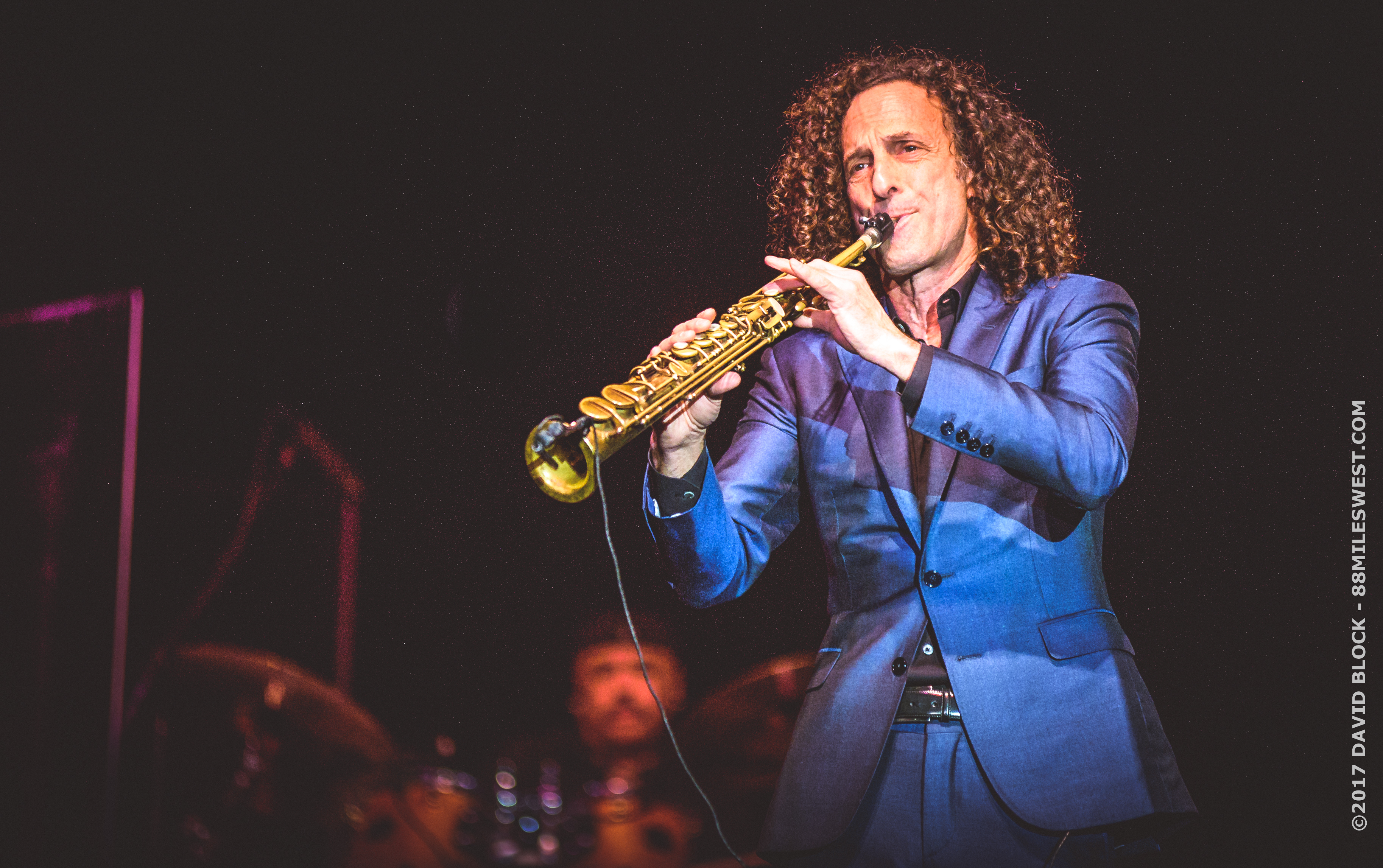The photograph captures the famous musician Kenny G performing with his unique brass, gold-colored instrument, which resembles a hybrid of a saxophone, clarinet, and flute. He is dressed in a dark blue suit, buttoned with a black button, accompanied by matching blue pants and a black shirt underneath. Kenny G's distinctive long, curly brown hair cascades over his shoulders as he intensely focuses on playing his instrument, blowing into it and manipulating it with his fingers. A wired microphone is attached to the end of his instrument, with the wires trailing down to the bottom of the image. The background is predominantly dark, with a black backdrop that accentuates the performers. Behind Kenny G, a drummer is partially visible, seated behind his drum set. White text runs vertically along the side of the photo, reading "© 2017 David Block, 88mileswest.com". The overall setting suggests an intimate concert atmosphere, highlighting the concentrated expression on Kenny G's youthful face as he passionately plays his music.